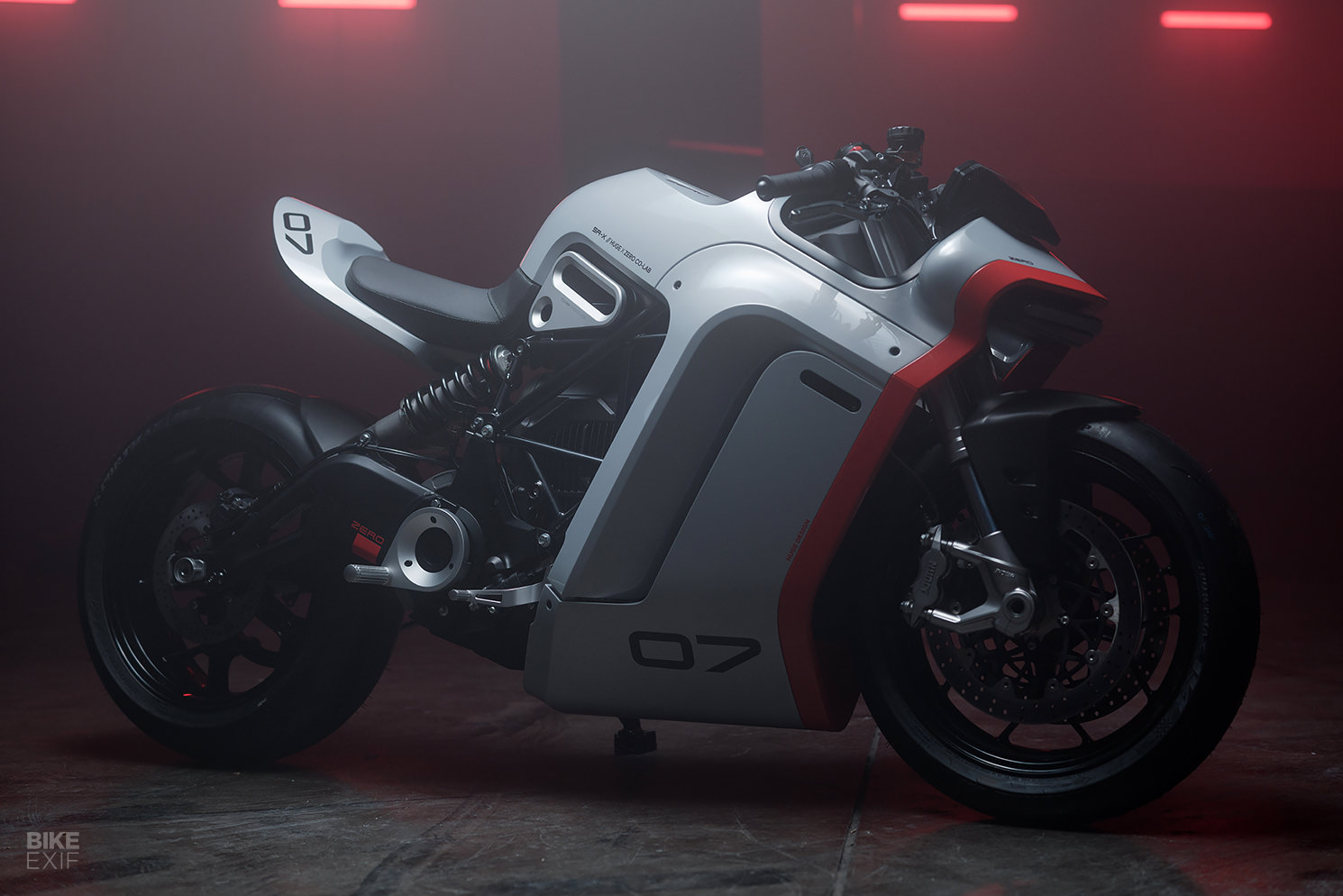This image features a photograph, or a computer-generated image, of a futuristic, compact street-style motorcycle. The setting is a dark room with a wall illuminated by horizontal red lights, casting a red glow across the scene. The motorcycle, positioned with its front facing right, has a sleek gray body with black tires, the rear one being slightly smaller. The bike boasts a silver plate on the rear fender and the bottom, both of which display the number "07". The design is highly modern and non-traditional, with a distinctive short body and black gear and suspension components. A red border frames the upper part of the bike. It rests on a gray tiled floor, which reflects the motorcycle slightly. In the bottom left-hand corner of the image, the word "Bike XIF" is noticeable.